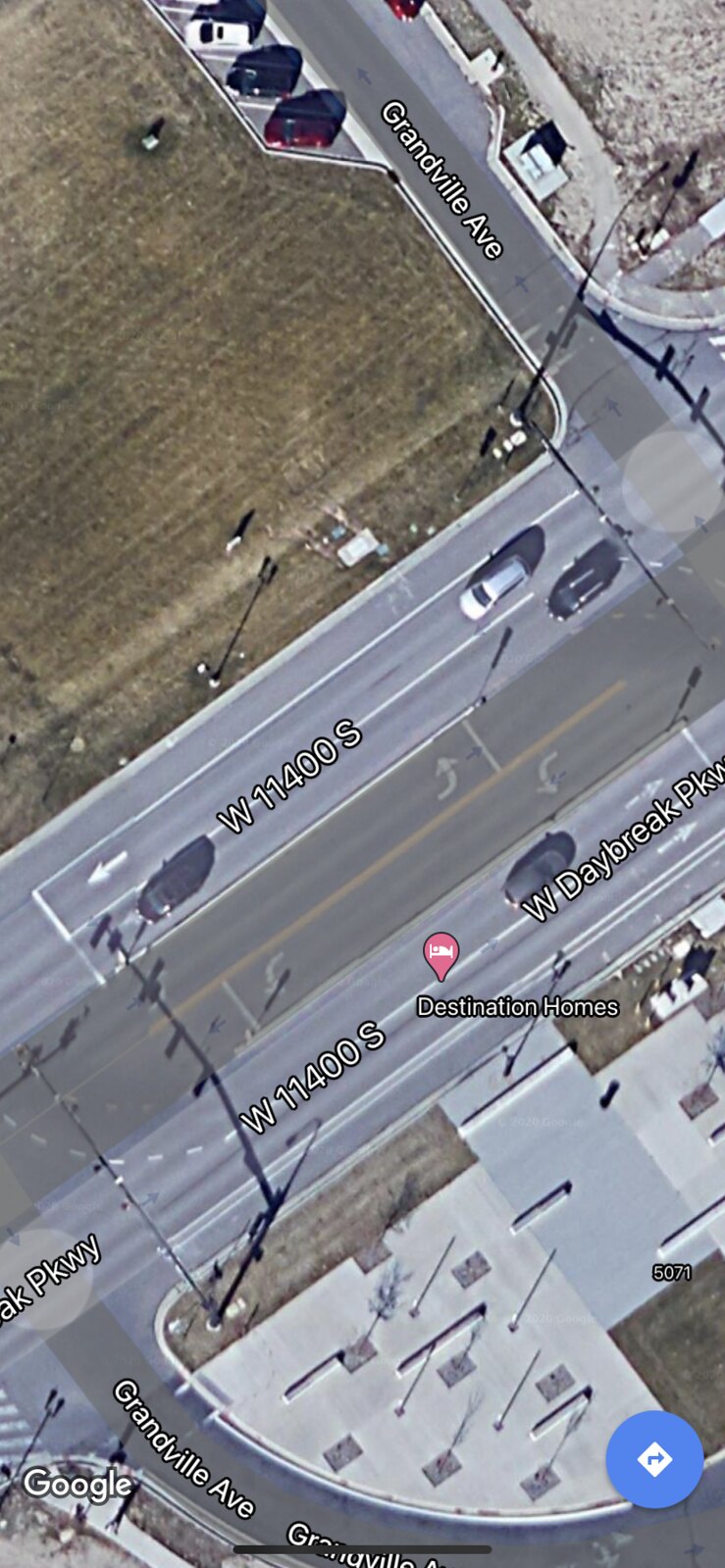This detailed color image appears to be a vertical screenshot from Google Maps, displaying an aerial view of a city intersection covered in various roads and landmarks. Prominently marked in white text, Granville Avenue appears twice—first from the top center extending down to the right edge and curving into a loop that re-emerges at the bottom center. Another major street, labeled W11400S, runs diagonally from left to right across the middle of the image. There's an additional road, West Daybreak Parkway, which runs parallel to W11400S and is partially obscured by the edge.

In the lower right-hand corner, the name "Google" is noted in white letters, reinforcing the map's origin. At the image's top-left, a green grassy area can be seen. Towards the bottom right corner, there's a cluster of buildings, including an office building labeled "Destination Homes" marked by a red pin.

Within the street network, cars in various colors, including white, black, and red, populate both the parked areas along Granville Avenue and the moving lanes of W11400S and West Daybreak Parkway. The intersection includes notable features such as utility poles, traffic lights mounted on black poles, and smaller patches of green spaces dotted around the concrete jungle.